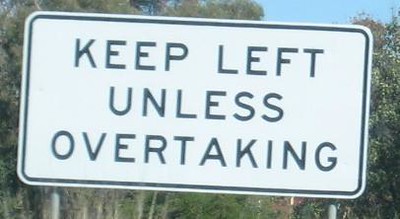The image is a detailed view of a highway sign prominently displayed against a natural backdrop. The sign is a large white rectangle with a black border, mounted on two silver metal posts, one on each end. It bears the instructions, "KEEP LEFT UNLESS OVERTAKING," written in bold black capital letters. The sign appears to be slightly tilted, with its left side raised higher than the right. Surrounding the sign are trees and bushes in varying shades of muted green, with a light blue sky visible in the background. The greenery appears somewhat dull, possibly due to fog or low image quality, adding a slightly hazy effect to the scene. The focus of the image is largely on the sign, with very little of the surroundings visible, emphasizing the sign's importance and presence.